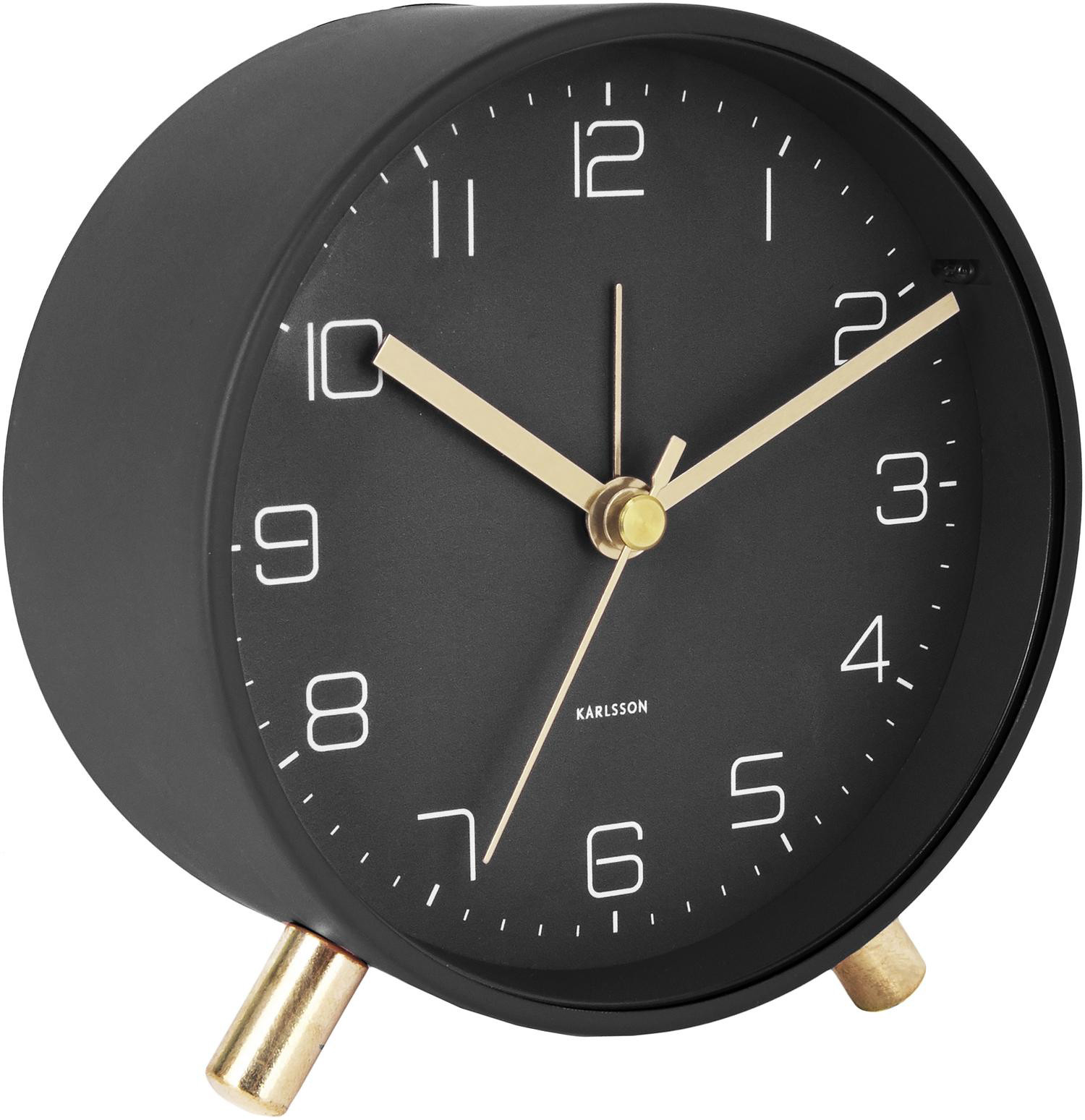This image features a classic black alarm clock, prominently displayed against a stark white background. The clock boasts a traditional round face with bold white numbers and minute markers contrasting against the black backdrop. The brand name "KARLSSON" is elegantly inscribed in white, just above the number 6. The clock's brass elements add a vintage charm—the hands (including an old-fashioned alarm hand fixed at 12) and the center circle are made of brass, as are its short, cylindrical legs. The overall composition and lack of other objects suggest the image could be from a product catalog, showcasing the clock in striking detail from a slightly angled perspective.